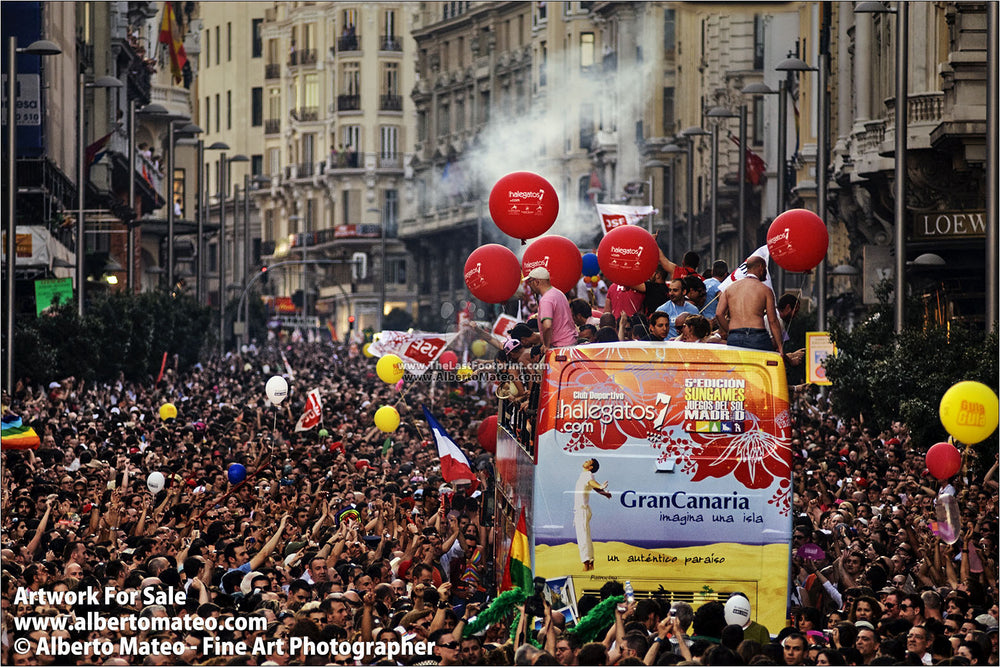In this colorful and bustling scene of what appears to be a gay pride parade in a densely packed Latin American city, thousands of people crowd the streets, surrounded by a backdrop of run-down, white and gray stone or brick buildings. The left side showcases buildings elevated on stilts, casting dark shadows underneath. Among the sea of people, many hold up various objects, including yellow, white, and pride flags, along with numerous red and white balloons. Central to the image is a luxurious double-decker tour bus adorned with vibrant advertising featuring Spanish writing, including "Gran Canaria", in hues of red, orange, yellow, and gray.

On top of the bus, a predominantly male group stands, some grasping five prominent red balloons, while others enjoy the elevated view. Notably, a man clad in a white shirt and pants, stands to the left of the bus's center, bending slightly backwards with his arms arched behind him, gazing skyward. The festive crowd surrounds the bus almost entirely, their arms raised in jubilation, filling the air with an atmosphere of celebration and unity. The city street is lined with historic multi-story buildings and dotted with streetlights and small trees, adding to the vibrant yet run-down Latin American charm of the scene.